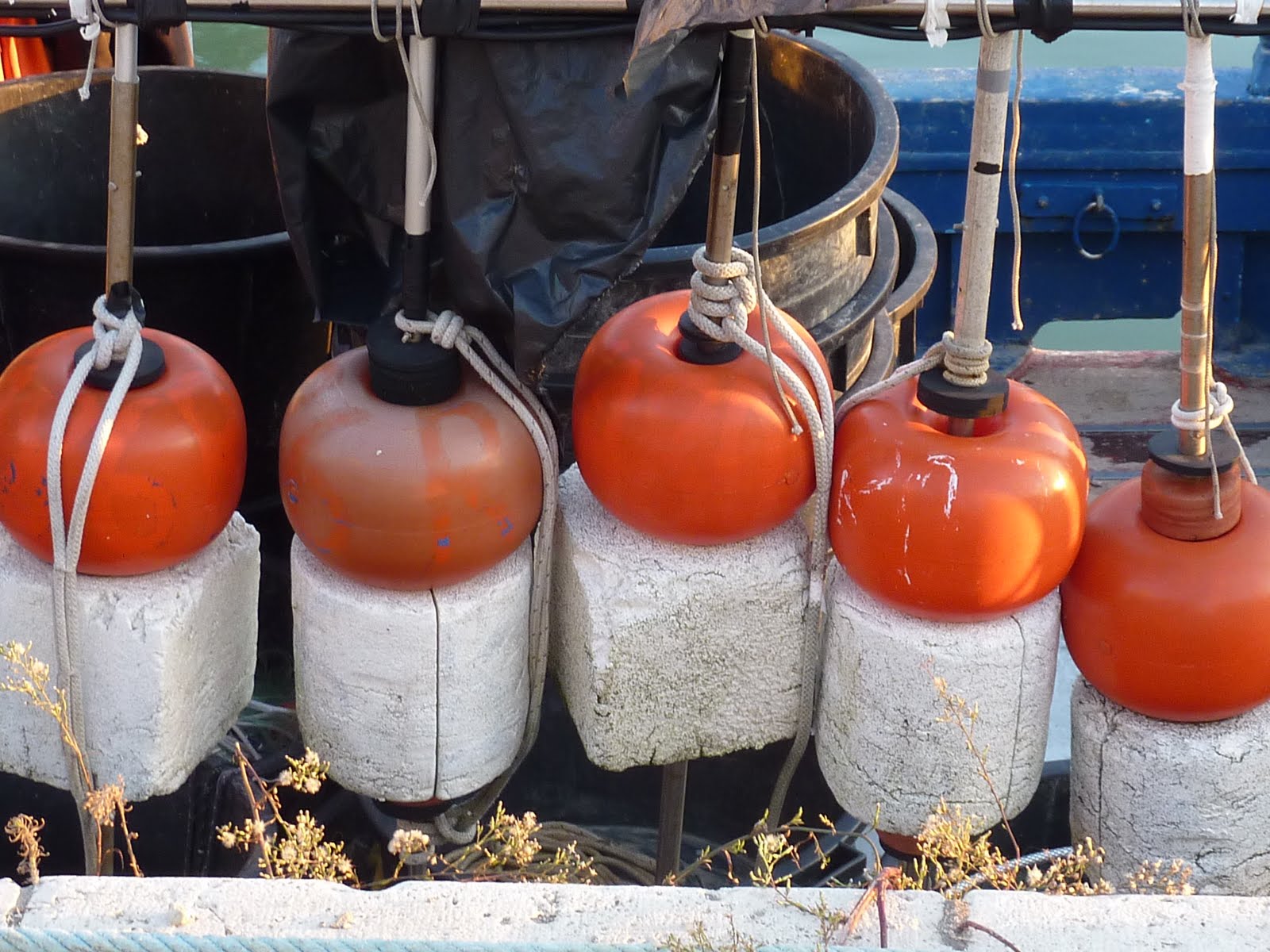The image captures a set of five aged buoys, each featuring a white base that is either square or circular and topped with a round, pumpkin-like, red-orange ball. These weathered buoys, all scratched and discolored, are suspended vertically from a horizontal rod, with ropes tied around their bases. The setting appears to be either a boat or dock area, evident from the presence of two large, dirty plastic containers and a black plastic bag hanging in the background. Additionally, to the right, there's a blue box with a handle. The natural lighting enhances the details of the buoys, highlighting their timeworn texture and the dust accumulation, especially noticeable on one buoy where someone has traced their initials in the dust.